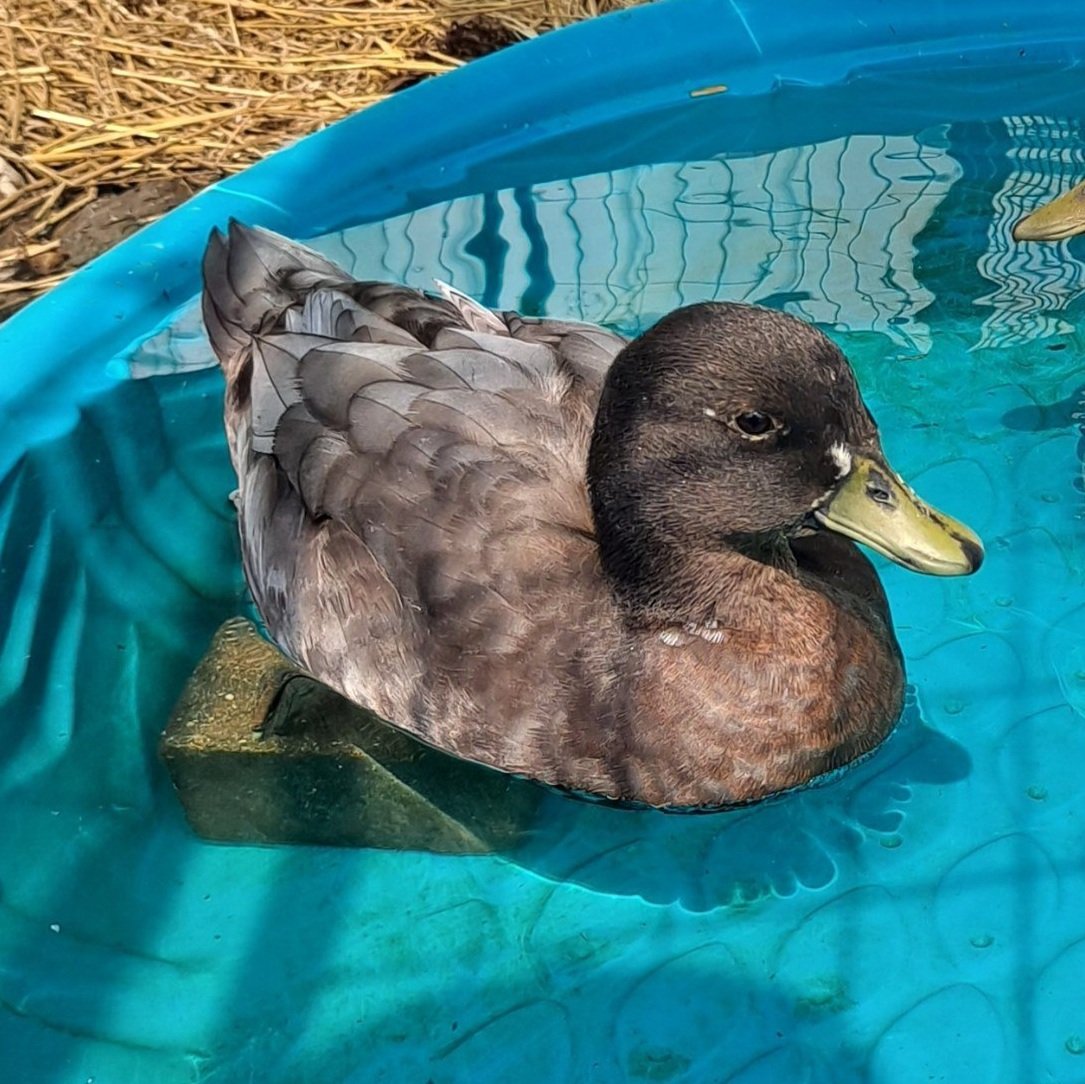The image captures a detailed scene of a blue plastic kiddie pool with a fish scale design on its bottom, situated in an outdoor setting that resembles a barn or farm due to the scattered tan hay surrounding it. This small pool, partially filled with water, hosts a vividly colored duck, primarily gray with a darker gray or black head, and a lighter gray to brown body. Its distinctive yellow-green bill is complemented by black eyes. There is a brick lying beneath the duck in the pool, possibly serving as a weight. The pool also contains some floating leaves and algae, adding to the rustic charm of the scene. Near the edge of the image, a second duck’s bill is visible, suggesting the presence of another duck. The background includes more hay and suggests a reflective surface, possibly from a nearby fence.